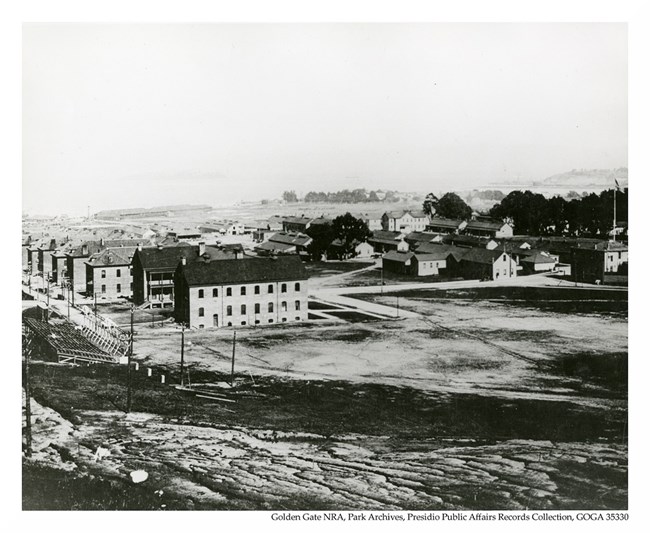This black and white photograph captures a serene village scene with rich historical significance, as evidenced by the caption "Golden Gate NRA Park Archives Presidio Public Affairs Record Collection GOGA 35330" at the bottom. The foreground features an expanse of very flat, ridged stone, transitioning into a neatly trimmed area of grass. A flattened plaza marks the central part of the town, which is populated by a series of rectangular buildings. 

On the left side, the buildings have black, sloped roofs that extend leftward off the image, and utility poles run parallel to this row. A metal grate protrudes from the field in this area. To the right, similarly shaped buildings are arranged perpendicularly to the first set. Trees dot the landscape with a gentle hill covered in a small forested area in the backdrop, while a larger, distant hill with scattered black tree-like splotches stands out further to the right. Intriguingly, a large boat is visible sailing past this distant hill, adding a dynamic element to the scene. The photograph’s stark contrast and repetitive architectural design contribute to its depiction of a typical albeit historically layered town.